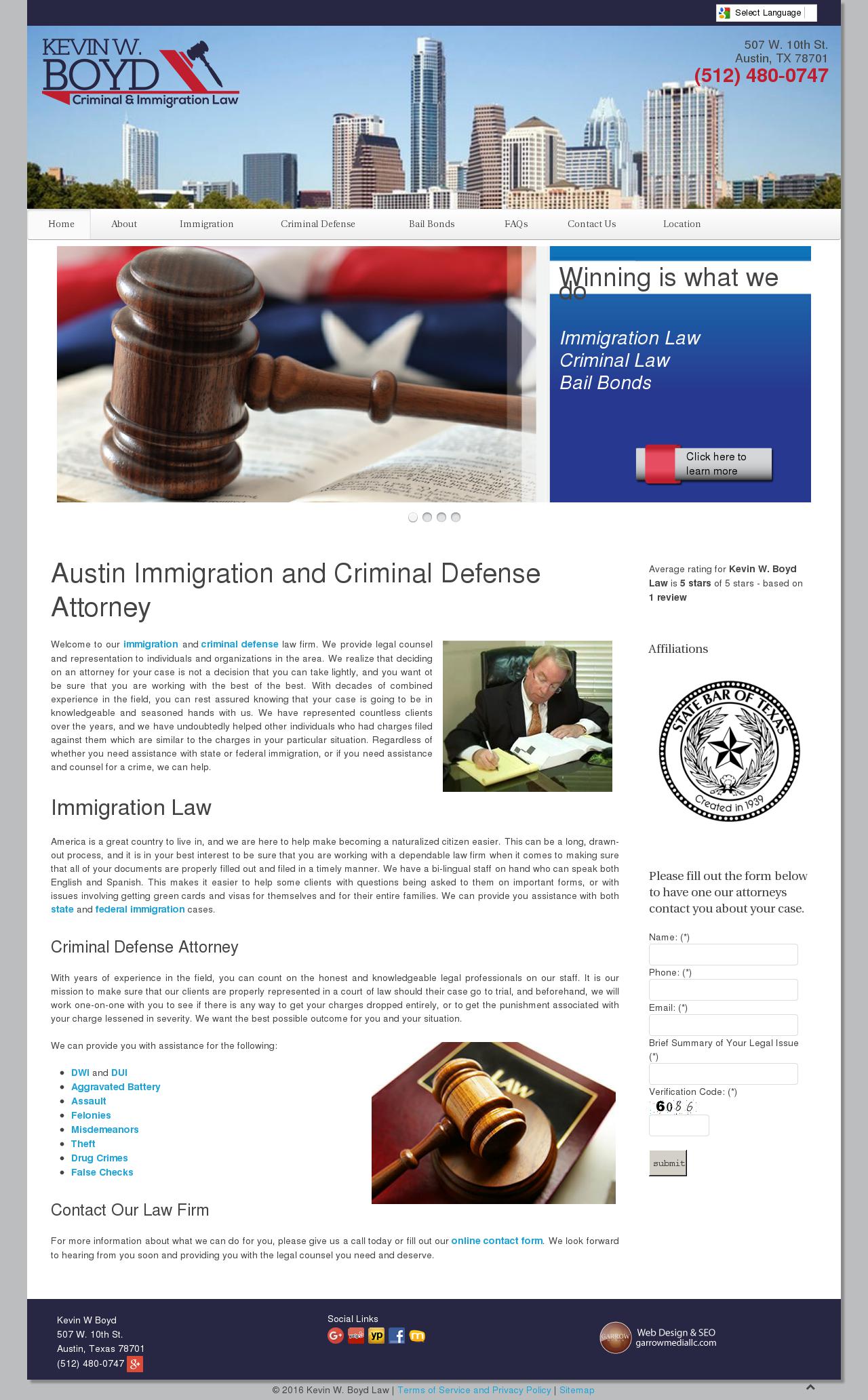Homepage for Kevin W. Boyd Criminal and Immigration Law

The webpage has a primarily white background accented by light gray borders along the bottom and sides. A dark navy blue rectangular banner spans the entire width at the top. In the upper right corner of this banner, there is a drop-down menu with black text for selecting a language. The header prominently displays "Kevin W. Boyd Criminal and Immigration Law" followed by a black gavel icon. To the far right, the office address is listed in black text: "507 West 10th Street, Austin, Texas 78701," and beneath that, in red text, is the phone number: "512-480-0747."

Below the banner, an image of a city skyline is featured, showing skyscrapers of varying heights, colors, and sizes set against a clear blue sky. Underneath the skyline image, a series of navigation links in black text is presented in a horizontal line: "Home," "About," "Immigration," "Criminal Defense," "Bail Bonds," "FAQs," "Contact Us," and "Location."

To the left, an open book with a dark brown wooden gavel set on it is displayed. To the right of this image, a blue square with black text reads, "Winning is what we [do]," followed by white text stating "Immigration Law, Criminal Law, Bail Bonds," with a prompt to "Click to continue."

The section beneath this header announces "Austin Immigration and Criminal Defense Attorney." Below this, a full paragraph describes the attorney's qualifications and services, accompanied by a photograph of Kevin W. Boyd. He is depicted as a middle-aged Caucasian man with light dirty blonde hair, wearing a black suit, white shirt, red tie, and glasses. To the right of his photograph is a list of affiliations, including the State Bar of Texas seal.

Further down, sections on "Immigration Law" and "Criminal Defense Attorney" each provide detailed paragraphs describing legal services in these areas. To the right, a contact form invites potential clients to fill in their "Name," "Phone," "Email," a "Brief Summary of your legal issue," a "Verification Code," and a "Submit" button.

Overall, the page is structured to provide comprehensive information about Kevin W. Boyd's legal services, with easy navigation and clear contact options for clients.